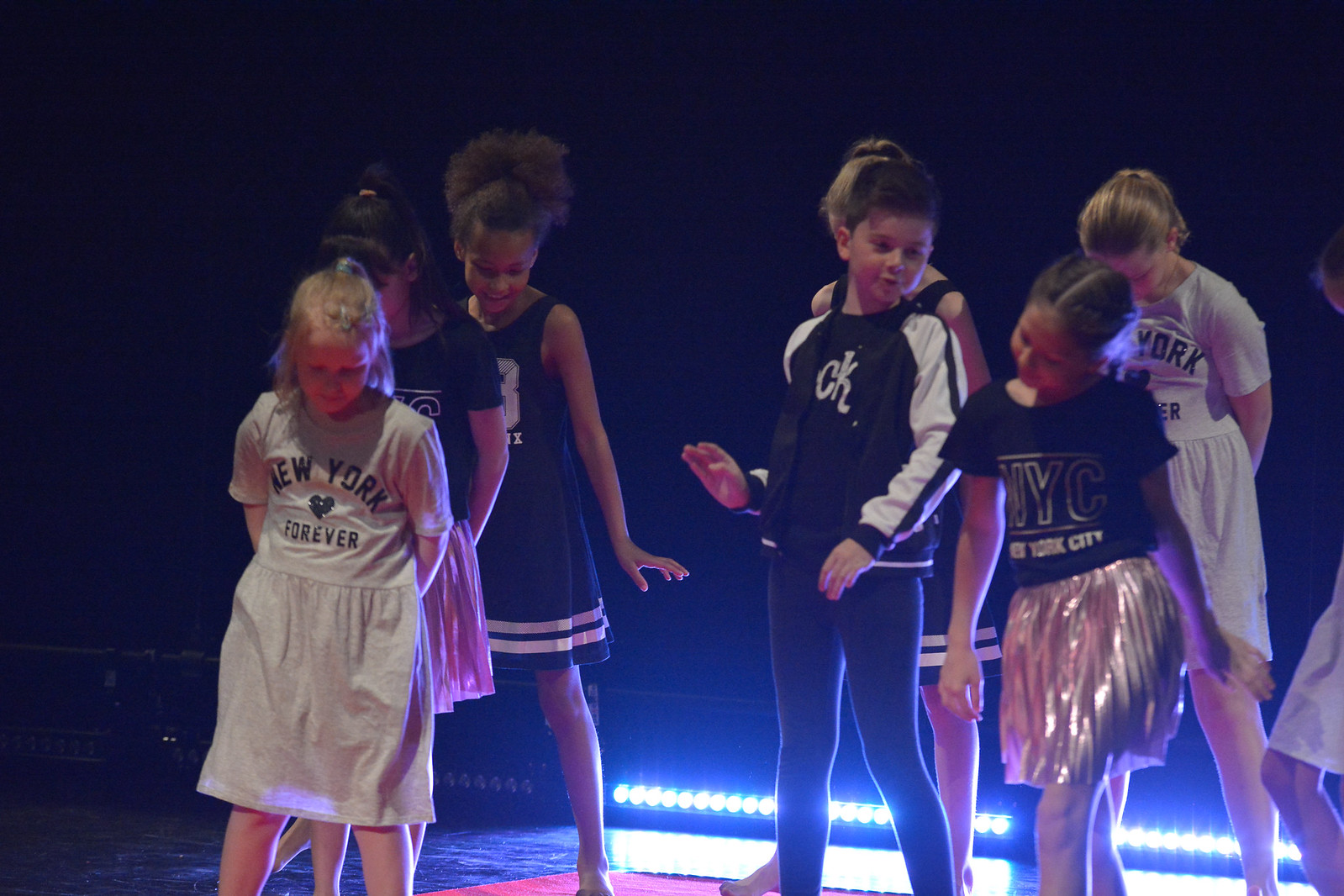The photograph captures a group of eight children, seemingly around six or seven years old, performing on a dimly lit stage. The backdrop is predominantly dark, with only the lower half of the stage illuminated by ankle-height string lights. The stage floor is primarily black with hints of a red carpet.

Among the group, a blonde girl stands prominently at the front, dressed in a white outfit—her top explicitly reads "New York Forever," accompanied by a heart graphic. Next to her is a small brunette girl wearing a black shirt inscribed with "NYC New York City" and paired with a gold skirt. 

Further back, a boy is dressed in black pants and a matching black jacket, suggestive of a sleek uniform or costume. The setting includes an LED light that significantly brightens the stage behind them, adding emphasis to their performance. Other children, including a black girl, mostly wear attire that hints at cheerleading or dance outfits, reinforcing the idea that this could be some sort of cheerleading or dance competition. The children’s expressions and coordinated clothing featuring New York themes suggest they might represent a New York-based team or group.